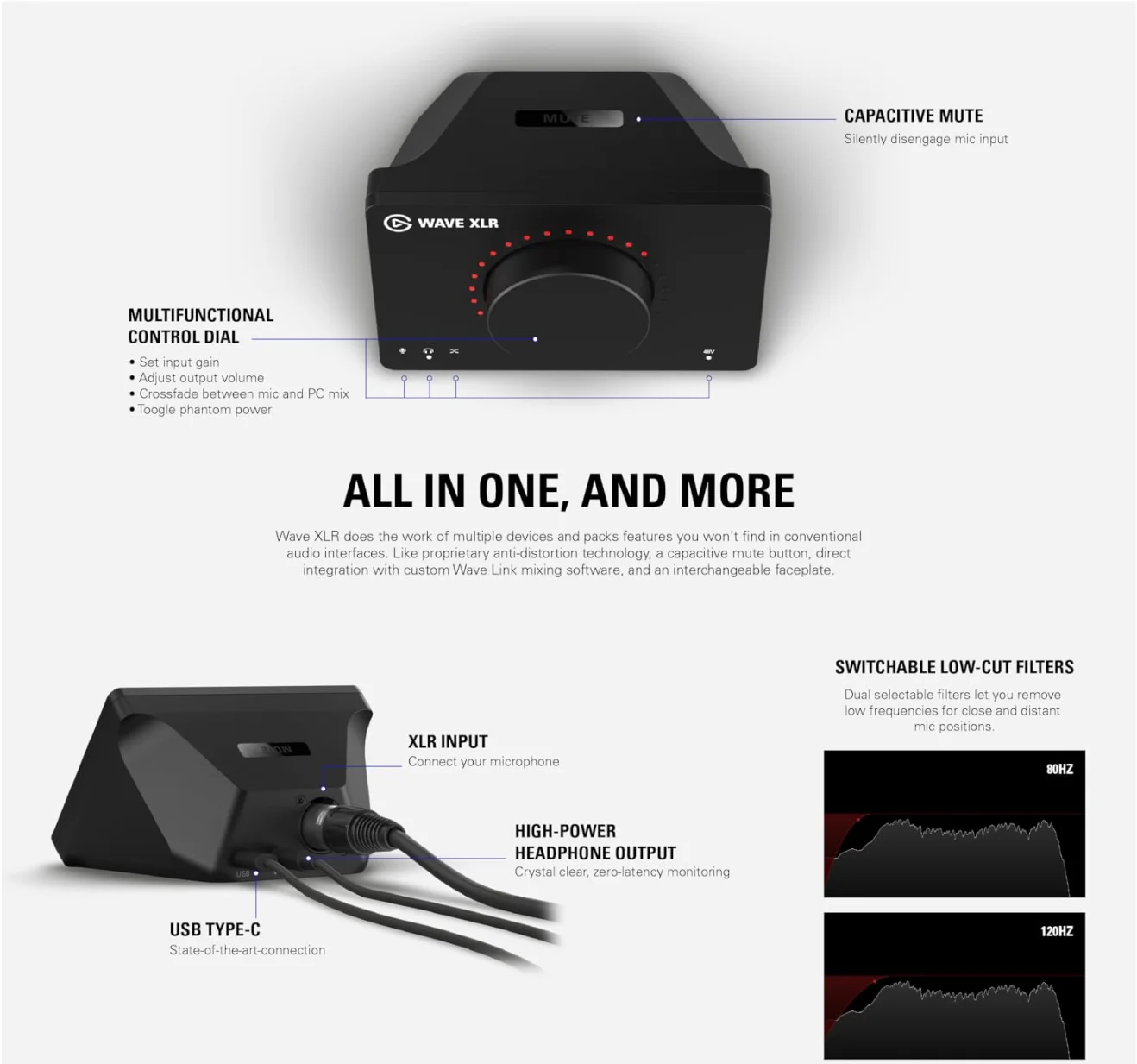This advertisement presents the WaveXLR, a versatile black audio interface designed for comprehensive mic control. The infographic prominently displays the sleek, rectangular black device featuring a multifunctional control dial encircled by red dots indicating varying levels of adjustment intensity. The dial facilitates setting input gain, adjusting output volume, crossfading between mic and PC mix, and toggling phantom power. Notably, it includes a capacitive mute button that allows for silently disengaging the mic input.

Highlighted in large text below the image, the slogan "All-in-One and More" emphasizes the multifunctional nature of the WaveXLR. The accompanying paragraph elaborates on its capabilities, detailing that the WaveXLR consolidates multiple device functions into one unit, boasting features like proprietary anti-distortion technology, direct integration with custom Wavelink mixing software, and an interchangeable faceplate.

Further imagery within the ad showcases the device's connectivity options. The back view illustrates the USB Type-C port, XLR input for mic connection, and high-power headphone output for zero-latency monitoring. Adjacent to this depiction, dual graphical displays in the bottom right corner explain the switchable low-cut filters available at 80 Hz and 120 Hz, useful for minimizing low-frequency noise across different mic placements.

Set against a white background, this advertisement efficiently communicates the WaveXLR’s comprehensive functionality and innovative features, making it an essential tool for anyone seeking high-quality audio management.